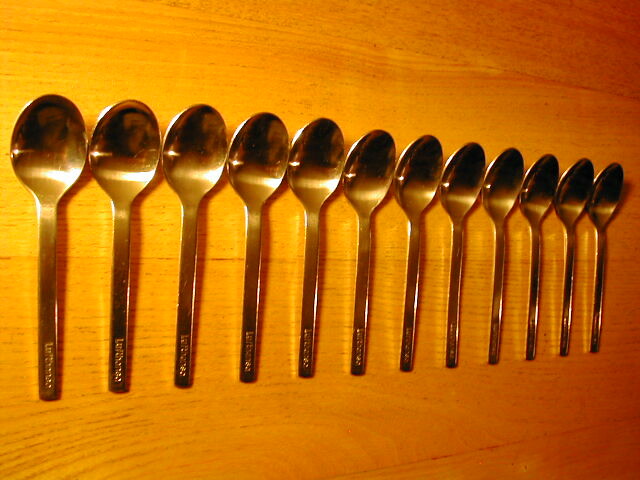The image features twelve silver spoons meticulously arranged in a straight row on a light honey-colored oak table. The perspective of the photograph, where the handles are oriented towards the bottom, seems to create an illusion of the spoons decreasing in size from left to right, although they may all be identical in size. The spoons have simple, elegant designs, with some subtle etchings or designs at the tips of their handles, though these details are not clearly visible due to the orangey light reflecting off their surfaces. This light gives the silver spoons a darker, warm hue, enhancing their visual appeal against the horizontal grain of the wood background.